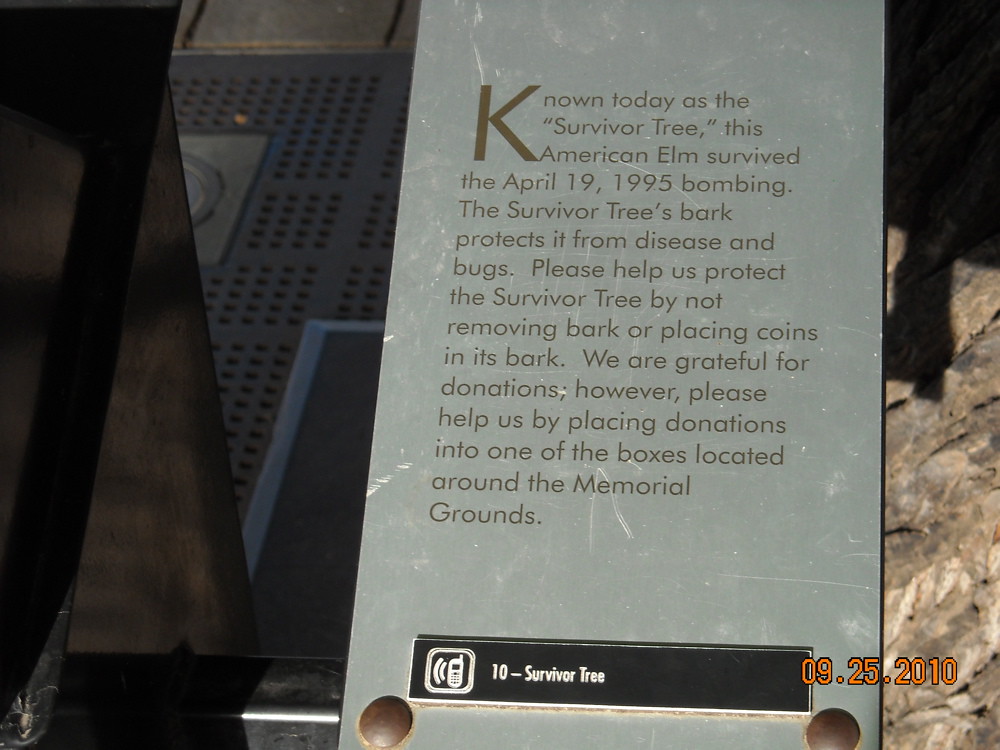The image shows a close-up of a light gray metal placard, bolted into another surface, with the following text written in brown letters: "Known today as the Survivor Tree. This American elm survived the April 19, 1995 bombing. The Survivor Tree's bark protects it from disease and bugs. Please help us protect the Survivor Tree by not removing bark or placing coins in its bark. We are grateful for donations. However, please help us by placing donations into one of the boxes located around the memorial grounds." In the lower section of the placard, there's a graphic of a phone accompanied by "10-Survivor Tree." The photo, taken on September 25th, 2010, has a mostly dark background and was presumably taken in Oklahoma City, where the historical significance of the Survivor Tree is rooted.